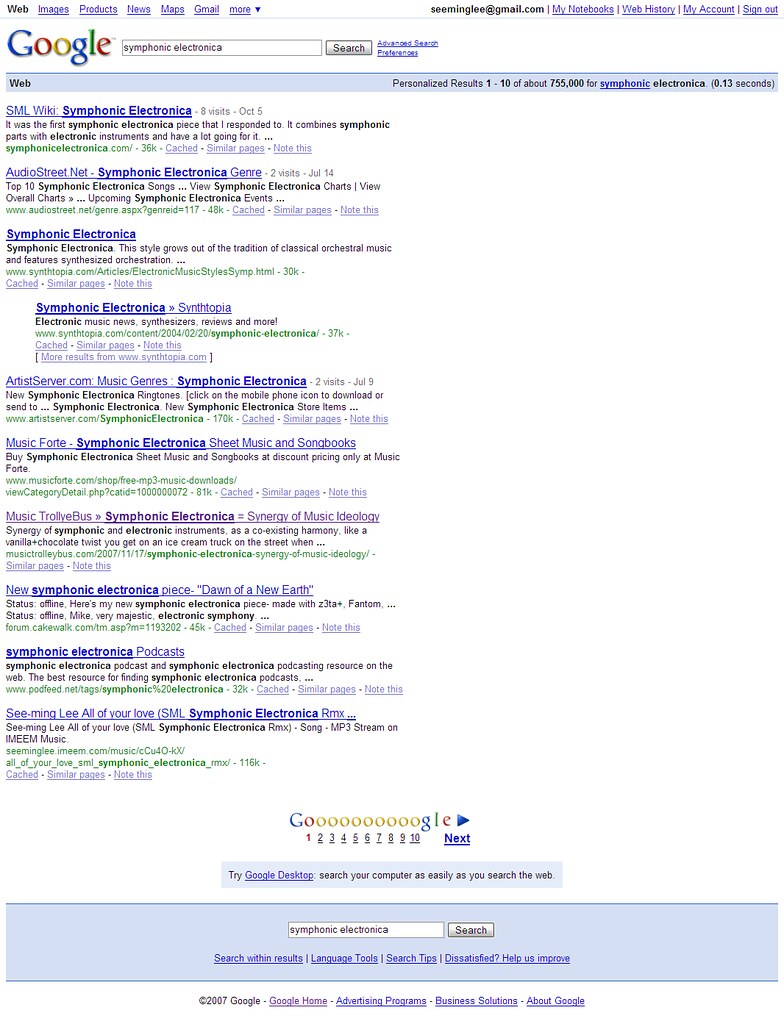This detailed caption describes an image of a Google search results page for "Symphonic Electronica":

"In the image, a Google search results page for 'Symphonic Electronica' is prominently displayed. At the top of the page, various categories are listed including Web, Images, Products, News, Maps, Gmail, and a dropdown menu labeled 'More.' The top-right corner features links to Gmail, My Notebooks, Web History, My Account, and a Sign Out option. Centered at the top, the Google logo is presented in its iconic blue, red, yellow, blue, green, and red color scheme, adjoining the search field.

Beneath the search field, a snippet of text from an online source, potentially the SML wiki, is visible. The text reads: 'Symphonic Electronica. It was the first Symphonic Electronica piece that I responded to. It combines symphonic parts with electronic instruments and has a lot going for it.'

The search results page shows 10 search results in total, each providing links and descriptions related to 'Symphonic Electronica,' offering an expansive overview of the topic. The page is a typical Google search layout, designed for user-friendly navigation and quick access to relevant information."